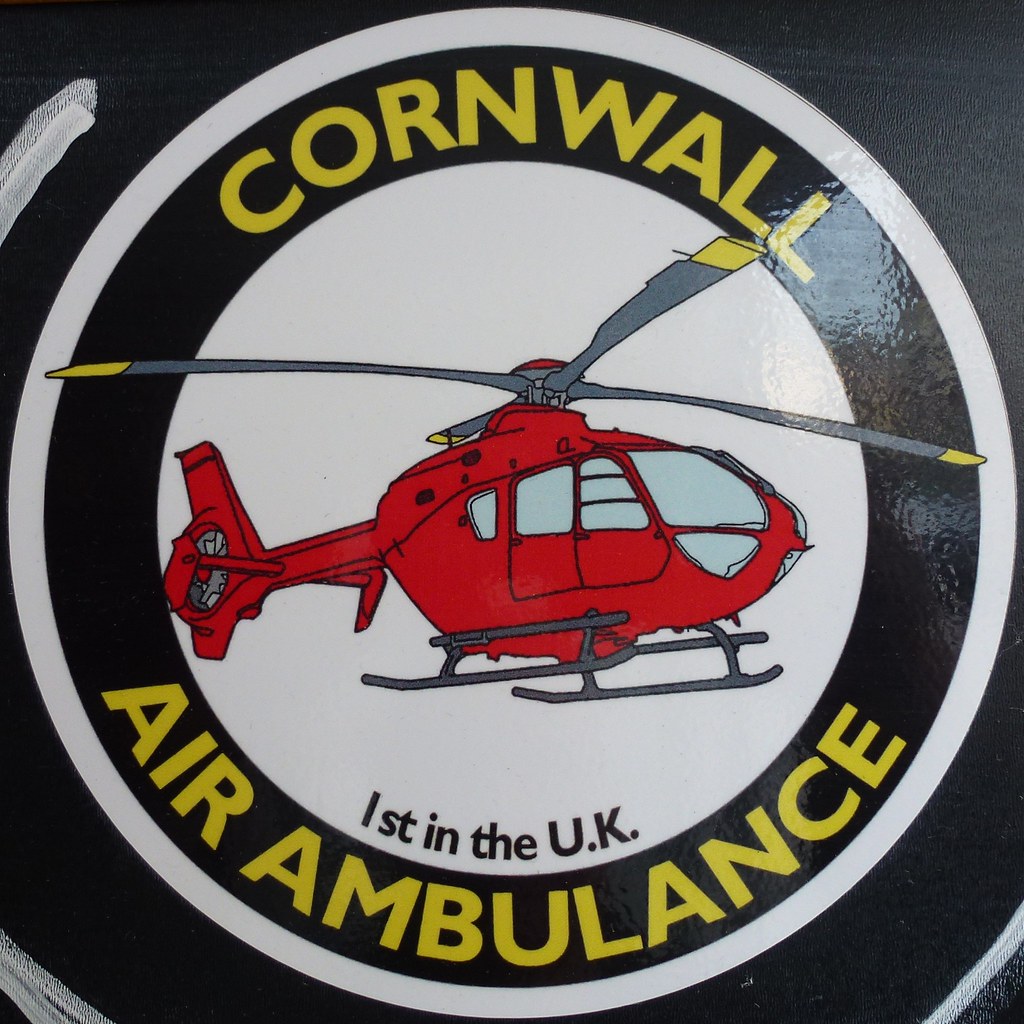The image showcases a detailed decal or sticker positioned on a black surface. The main feature is a large circular design, bordered by a thin white line and a black outline. Within this circle, the border features yellow text that reads "Cornwall" at the top and "Air Ambulance" at the bottom. The interior of the circle is filled with a white background, showcasing a red helicopter prominently at the center. The helicopter is detailed with dark gray propellers, which have yellow tips, and matching gray landing legs. The helicopter also features distinct windows and other external details. Below the helicopter, the text "First in the UK" is displayed in black. The edges of the decal seem to exhibit some white lines extending outward, creating a slight illusion of depth against the black surface. Overall, the sticker's vibrant colors and precise details make the design stand out clearly on its dark background.